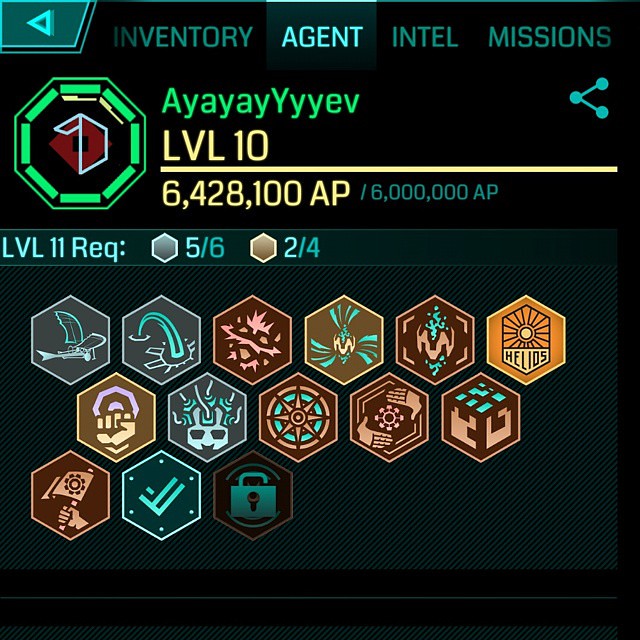This image is a detailed screenshot from a role-playing video game, showcasing a dark, black background with light green, illuminated text at the top, which reads like a menu. The menu includes the options: Inventory, Agent, Intel, and Missions, with the "Agent" tab highlighted. The top section displays a username, "IEIEIEIEF" at Level 10, with 6,428,100 AP (Action Points). The screen indicates that the next level requires 6 million AP, and the player currently holds 5 silver hexagons and 4 bronze. Below this information, there is a series of hexagon-shaped icons representing the player's earned badges. These icons are arranged in three rows towards the left-hand side: 6 icons in the top row, 5 in the second, and 3 in the third. The third icon in the second row is locked, marked by a padlock symbol. The other icons display various symbols such as a compass rose, a flying creature, a checkmark, Medusa, a pair of hands, a fist with a bullseye, a fish, a sun, and a flag. The graphic does not indicate the game's name.